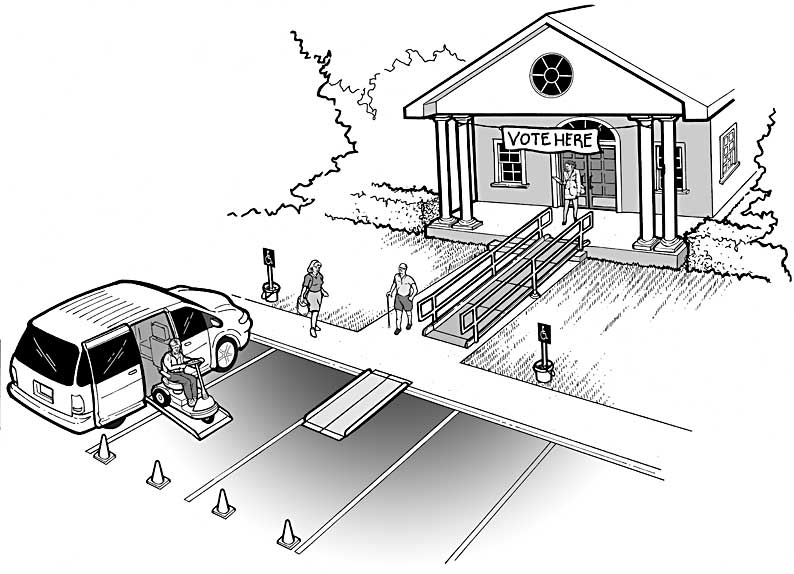This detailed black-and-white sketch depicts a voting site set in a classically styled, small building, possibly a church. The building features a triangular roof supported by columns and a circular window under the gable. A prominent banner reading "VOTE HERE" is tied to the façade above double wooden doors. Surrounding the building are trees and hedges, adding to its serene environment.

In the foreground, there's a small parking lot, partially obstructed by traffic cones, with a white van parked in one of the spaces. The van has a handicap-accessible ramp extended, and a man on a mobility scooter is emerging from it. Near the building, a clearly marked handicap ramp leads to the entrance. On the pathway in front of the building, a woman in a white dress stands by the doors, while a man with a cane and another woman navigate the sidewalk—either approaching or leaving the voting site.

The scene combines elements of accessibility with classical architectural beauty, effectively illustrating a welcoming and inclusive environment for voters.